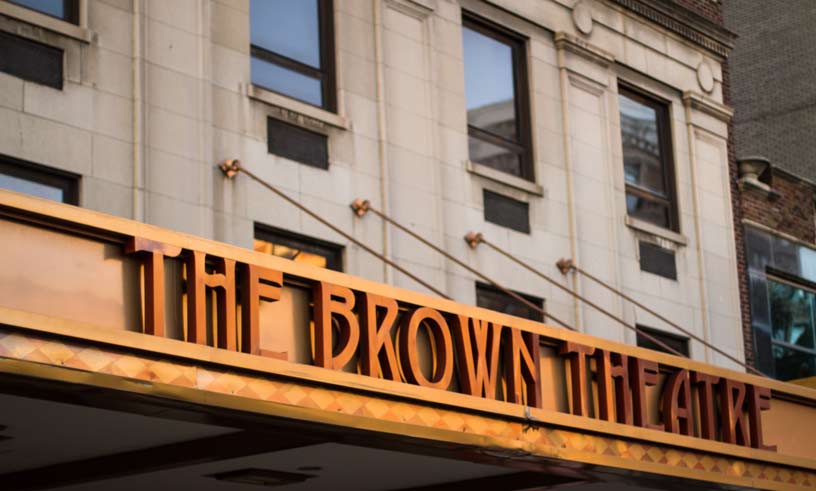This photograph captures the historic Brown Theater, an architectural gem likely constructed around a century ago. The focal point is a prominently displayed bronze-colored marquee with art deco or modernistic lettering spelling "The Brown Theater." This sign, mounted inside a shadow-box-like frame, is secured with cables to the whitewashed stone façade of the building. The ornate trim and distinctive 3D letters lend an air of elegance and nostalgia to the scene. The structure itself features multiple large windows, reflecting a serene blue sky and hinting at the surrounding urban environment. In the upper right corner, portions of two additional brick buildings are visible, adding depth and context to the location, which might be in New York or somewhere in the northeast. The photo suggests an overcast day, enhancing the timeless and stately ambiance of this iconic landmark.